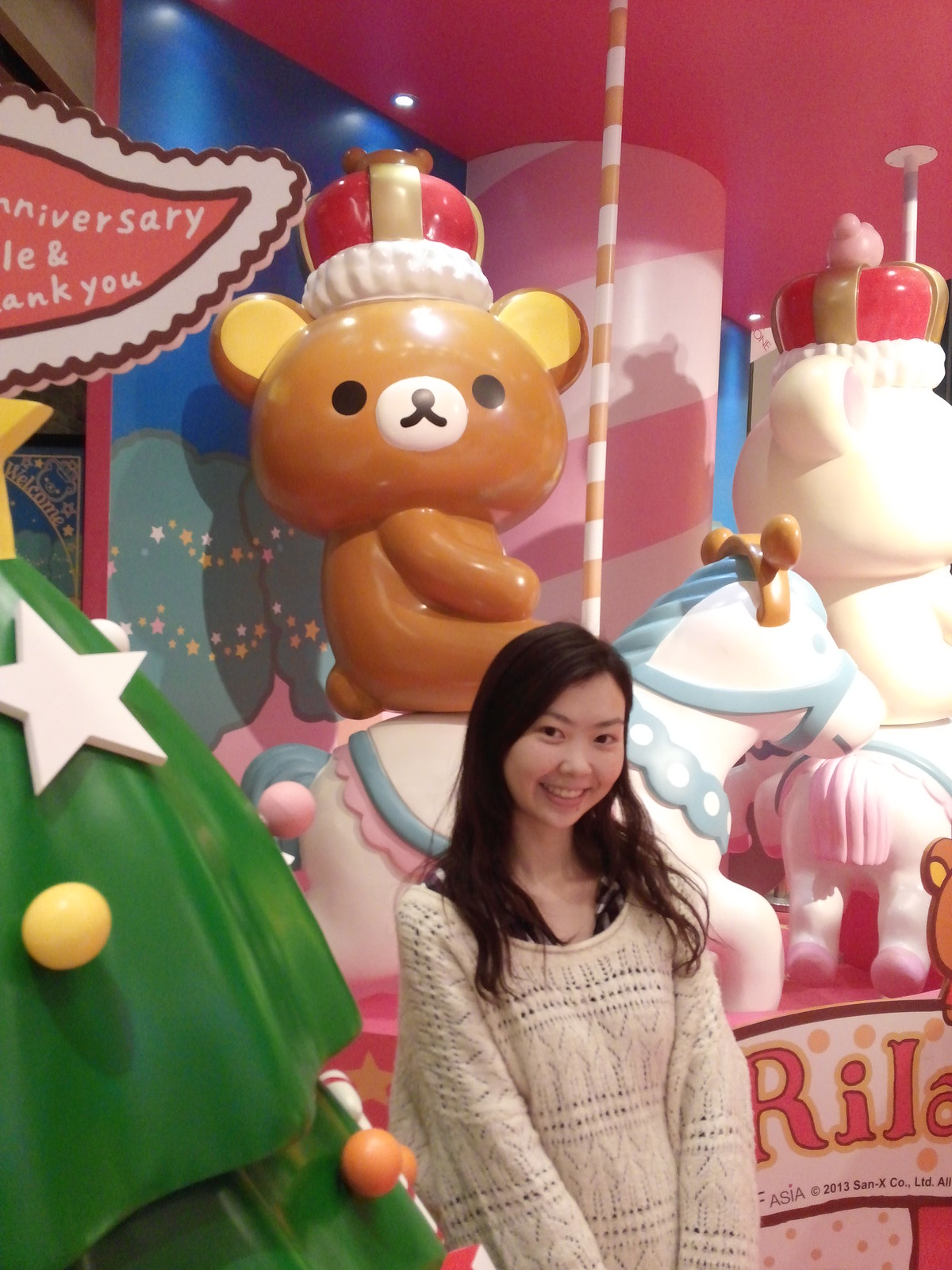In this picture, we see a young Asian girl, possibly around 15 years old, with long, black hair cascading over her shoulders and a cheerful smile, showcasing her teeth as she looks directly at the camera. She is wearing a white or milky-colored long sleeve sweater with subtle lines and pale colors, and underneath, she has a black and white checkered garment. Standing beside her is a decorated plastic Christmas tree adorned with red, orange, and white star-shaped ornaments, and a yellow star at the top. The backdrop features a merry-go-round with white poles striped in pink and red, where a large brown bear with a red and white hat sits on a blue, pink, and white horse. Another bear, which is white and adorned with a crown, can be seen just in front of the brown bear. Behind the girl, the partially visible words "Anniversary" and "thank you" appear along with "Rilla" and "Asia" written in red on a white background.